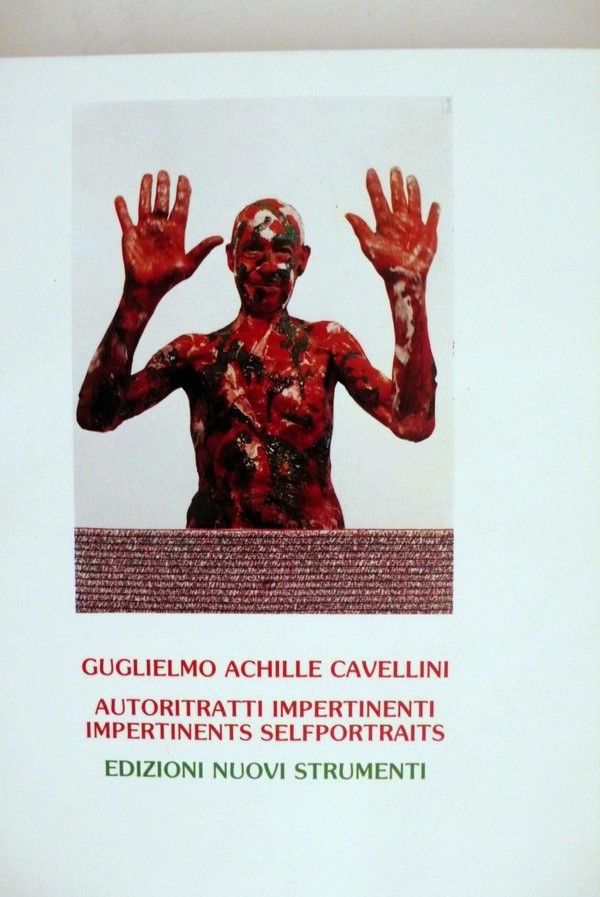The image depicts what appears to be a book cover, possibly also serving as a poster or promotional flyer. It features a bald man holding both hands up, palms facing outward with fingers somewhat spread apart, in a gesture reminiscent of surrender. He is covered in a mix of red, black, and white paint, giving him a gruesome, yet intriguing appearance. Despite his unsettling appearance, he is smiling with his mouth closed, directing his gaze toward the viewer. The background is plain white, and only the upper half of the man's body is visible, as a wall in front of him cuts off the view from the waist down. At the bottom of the image, there is a text in Spanish, followed by the name "Guglielmo Achille Cavellini" and the phrase "Autori trati impertinenti. Impertinent self-portraits. Edizioni nuovi strumenti," suggesting that this might be the cover of an art book or a promo piece for the said artist. The combination of the man's expression, the vivid paint, and the detailed text at the bottom creates a striking and memorable visual.